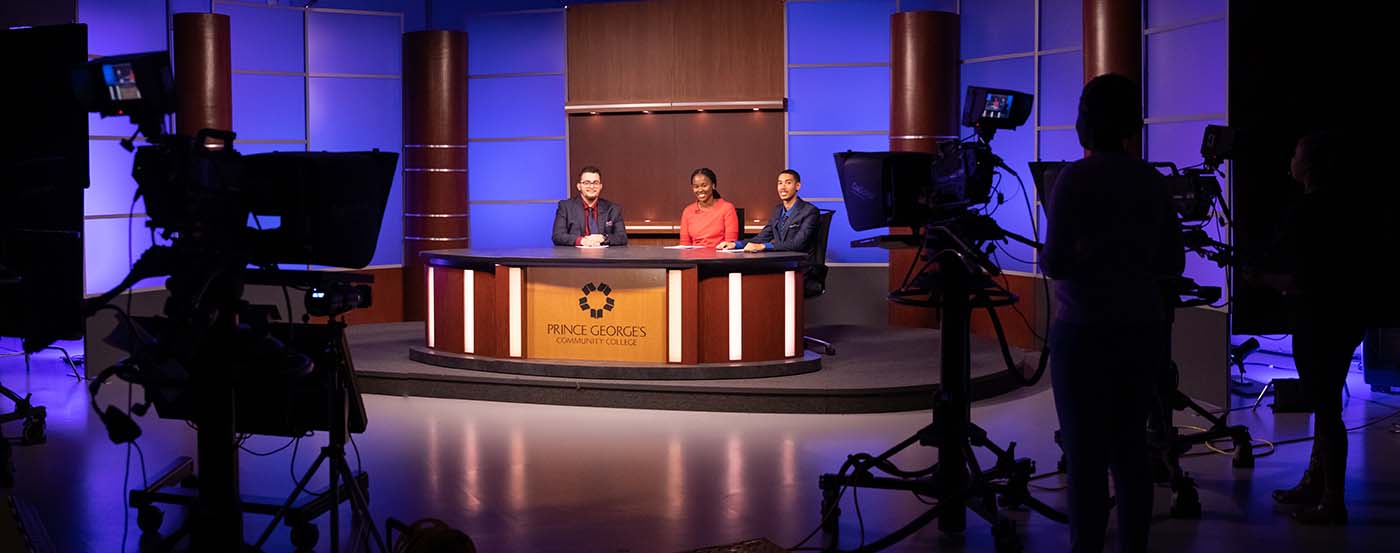The photograph captures a behind-the-scenes moment of a news broadcast at Prince George's Community College. Taken from the production side inside the television studio, the image shows the dark silhouettes of studio cameras and cameramen positioned at the right and left foreground, focusing on the brightly lit news desk at the center. The news desk, an ovular design made of brown and white wood with a flat black top, features the college's logo—a round circle with five stylized dark petals—and the text "Prince George's Community College." Seated at the desk are three news anchors: a woman in a long-sleeved top situated in the middle, flanked by two men in dark suit jackets. The newsroom studio is adorned with big brown pillars along the walls and large deep blue panels, including a prominent brown panel behind the news anchors that adds a touch of elegance to the set. The detailed setup captures both the technical and aesthetic elements of a professional broadcasting environment.